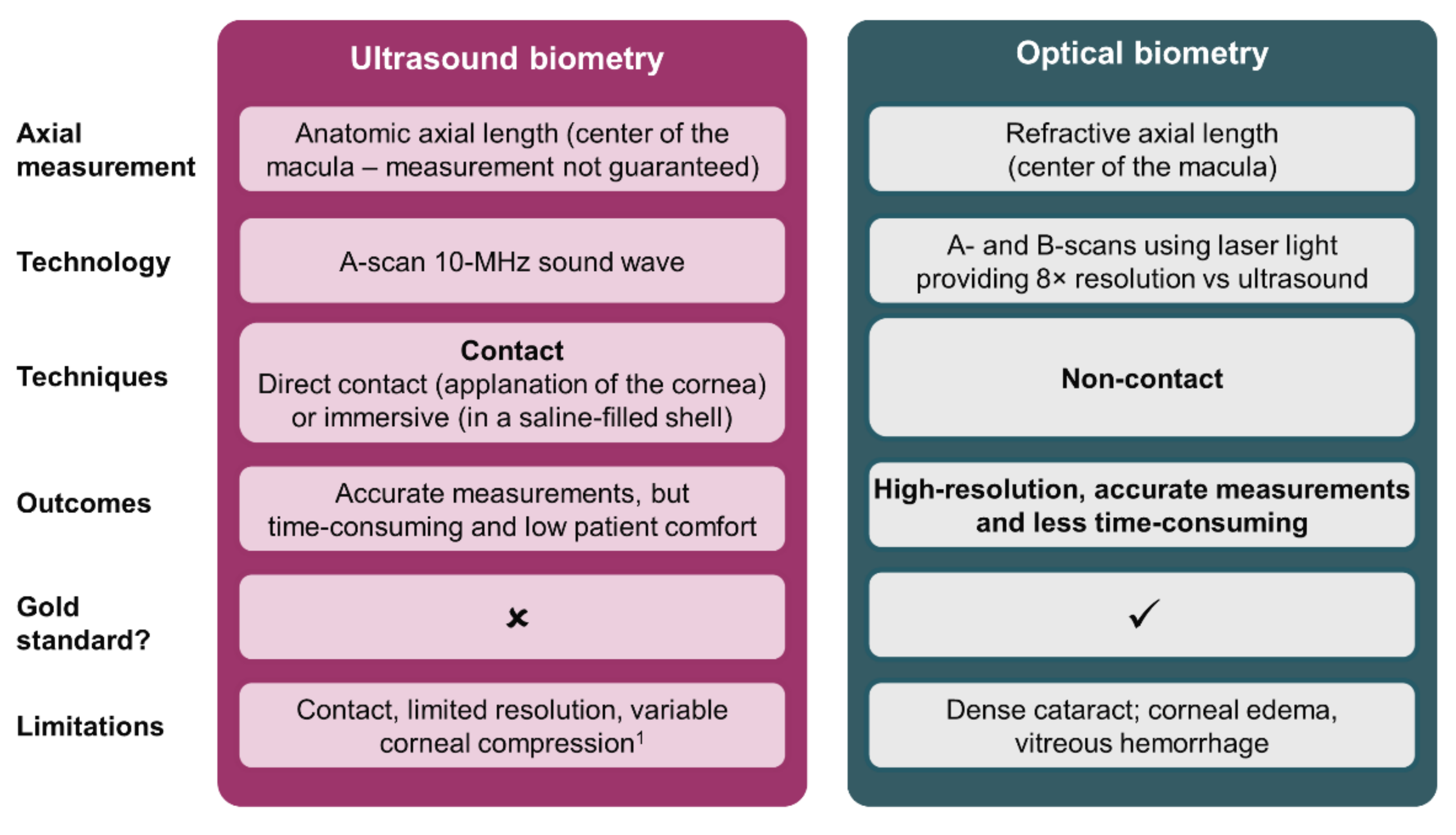The image is an informative slide comparing two methods for measuring the macula of the eye: ultrasound biometry and optical biometry. This comparison is organized in two vertical rectangles—purple on the left for ultrasound biometry and gray on the right for optical biometry. Each column lists attributes such as axial measurement, technology, techniques, outcomes, gold standard status, and limitations.

**Ultrasound Biometry (Purple)**:
- **Axial Measurement**: Anatomic axial length, with the center of the macula measurement not guaranteed.
- **Technology**: Uses a 10 MHz sound wave scan.
- **Techniques**: Contact-based, involving direct contact, either through applanation of the cornea or immersion in a saline-filled shell.
- **Outcomes**: Provides accurate measurements but is time-consuming and offers low patient comfort.
- **Gold Standard**: No.
- **Limitations**: Includes the necessity of contact, limited resolution, and variable corneal compression.

**Optical Biometry (Gray)**:
- **Axial Measurement**: Refractive axial length, with precise center of the macula measurement.
- **Technology**: Incorporates A and B scans using laser light, offering 8 times the resolution of ultrasound biometry.
- **Techniques**: Non-contact.
- **Outcomes**: Yields high-resolution, accurate measurements and is more efficient and comfortable for the patient.
- **Gold Standard**: Yes.
- **Limitations**: Affected by dense cataracts, corneal edema, and vitreous hemorrhage.

The slide effectively compares these two technologies to determine which provides better diagnostic results with minimal patient discomfort.